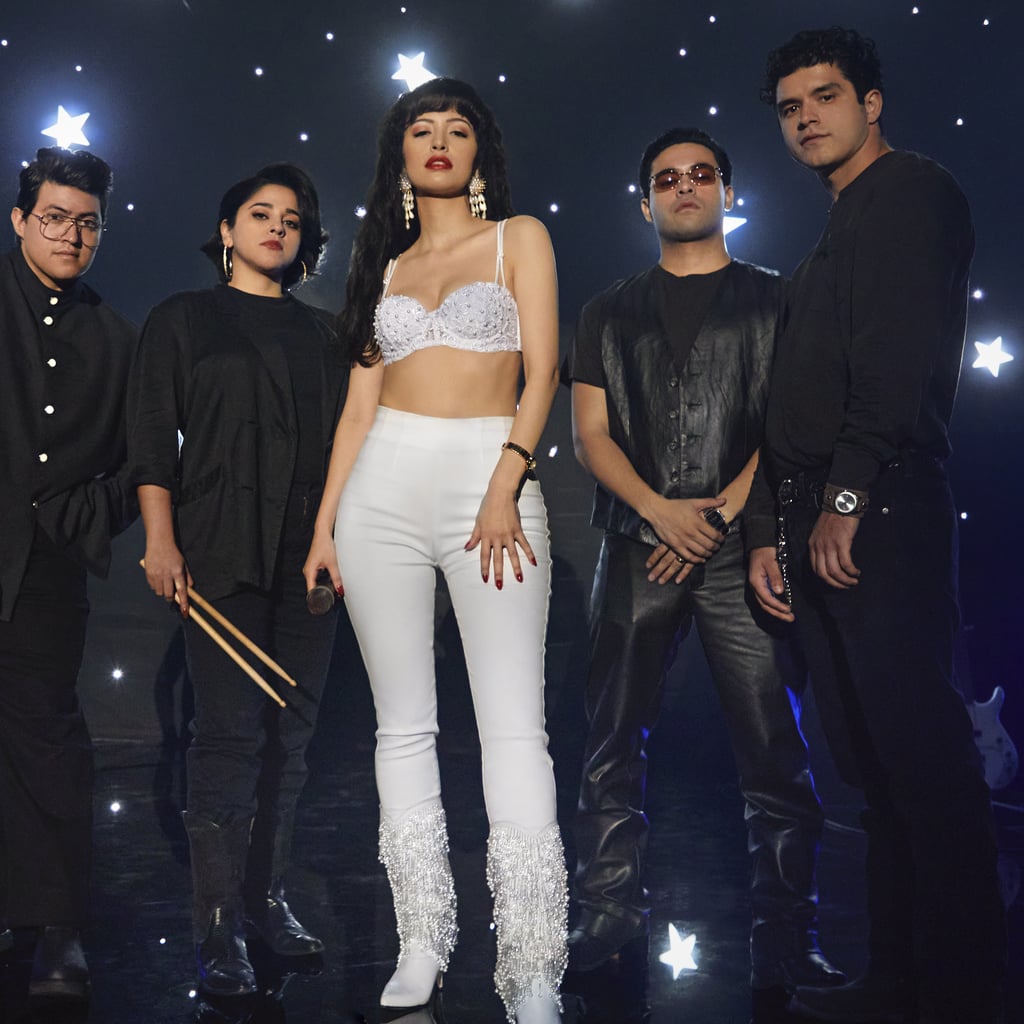In this dynamic stage photograph, the central focus is a striking female singer dressed in a dazzling white ensemble reminiscent of Tex-Mex icon Selena. Her outfit consists of tight-fitting white pants and knee-high white cowboy boots adorned with sparkling rhinestones. She also wears a matching white bra top encrusted with shiny gems, enhancing her glamorous stage presence. Complementing her glittering attire are long, dangly earrings, a black bracelet on her left wrist, striking red lipstick, and long, elbow-length black hair. 

The singer is flanked by four band members, all dressed in black. To her left stands a male band member and a female holding drumsticks, suggesting she might be the drummer. To her right are two more males, with one partially obscuring a guitar in the background. Together, they stand on a stage with a backdrop featuring many glowing white stars, evoking a celestial ambiance that highlights the group's performance setting. The composition of the photograph, the attire, and the equipment suggest this might be a tribute or a thematic performance, possibly echoing the style of the beloved Selena and her family band.